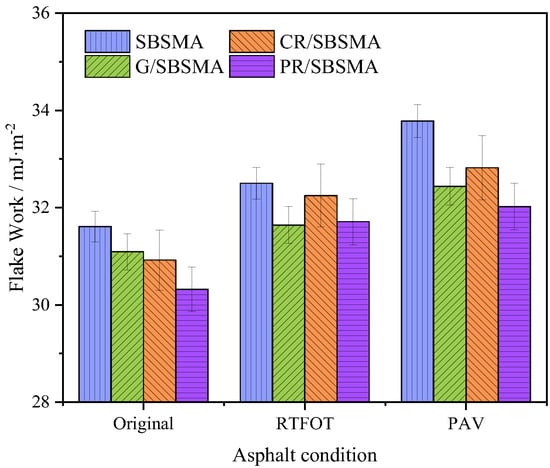The image features a detailed bar graph depicting asphalt conditions, with the x-axis labeled "Asphalt Condition" and divided into three sections: Original, RTFOT, and PAV. The y-axis, labeled "flakework/MJ·m⁻²," has a scale ranging from 28 to 36. Each section contains four colored bars—blue, green, orange, and purple—representing different materials as specified in the legend located at the top left corner. The blue bars stand for SBSMA, green for G/SBSMA, orange for CR/SBSMA, and purple for PR/SBSMA. The data shows that the bars in the "Original" section hover around 32, while those in the "RTFOT" section are slightly below 33. The "PAV" section has the tallest bars, with the blue bar reaching up to 34 and the others descending incrementally.